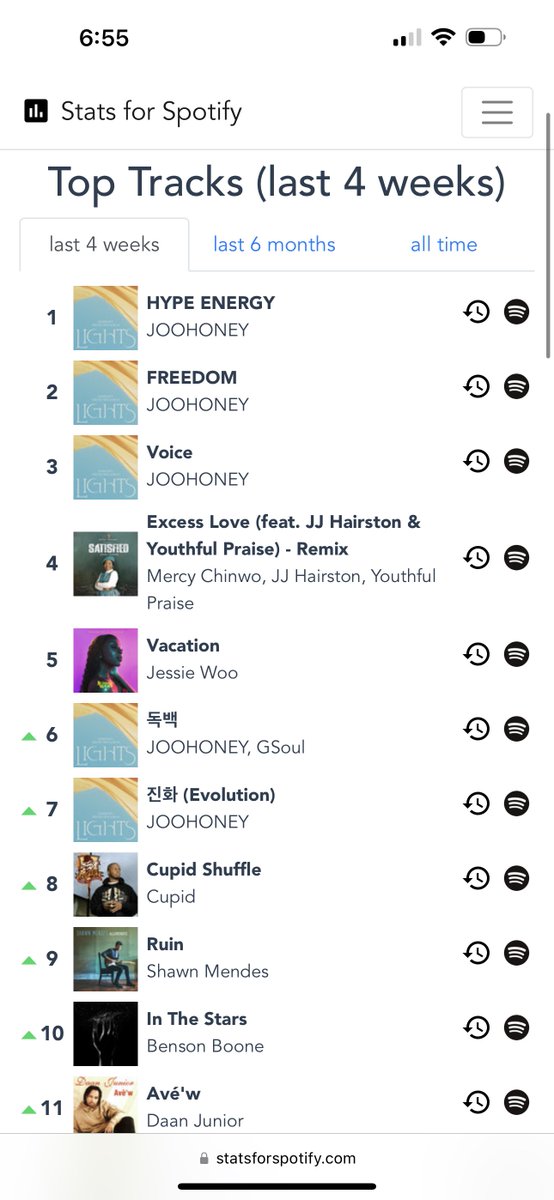The vertical image appears to be a screenshot from a smartphone. The background is predominantly white, similar to a computer screen. In the upper left-hand corner, the time is displayed in black text, showing 6:55. In the upper right-hand corner, there are icons representing the signal bar strength, Wi-Fi connection, and battery life.

On the left side, there is a small icon labeled "Stats for Spotify." Sliding to the right, there is a box containing three horizontal lines. Below a thin gray separator line, the text "Top Tracks - Last 4 Weeks" is written in bold black. Users have the option to select different time frames: "Last 4 Weeks," "Last 6 Months," or "All Time," with "Last 4 Weeks" highlighted.

The list beneath displays the top eleven tracks numbered consecutively from one to eleven. Tracks numbered six through eleven have an upward triangle indicating a rise in ranking. Next to each track number, there is a square featuring the album art followed by the track name and artist in bold black text. To the right of this information, there are several icons.

Track number one shows the following details: a picture with the text "Hype Journey" by "Joo Honey," followed by "Freedom" by "Joo Honey," "Voice" by "Joo Honey," and "Excess Love (featuring J.J. Hairston & Youthful Praise Remix)" by "Mercy Chinwoa, J.J. Hairston, and Youthful Praise."

The pattern continues for the rest of the list. At the bottom of the image, there is a web address followed by a thick black line.